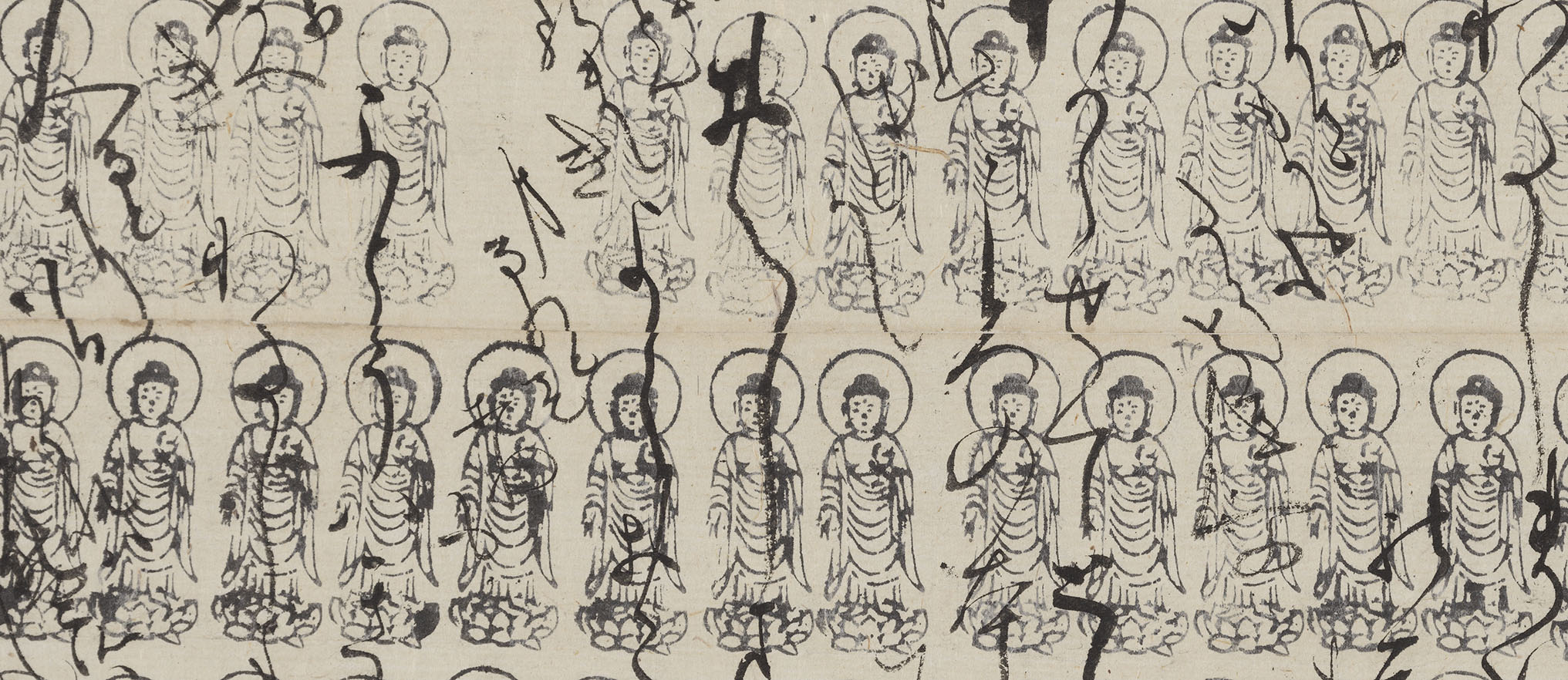The image depicts an artifact or piece of Asian art that is rectangular and horizontally oriented, measuring approximately 2.5 to 3 inches in height and 7 to 8 inches in width. The background is an off-white or light gray color, while the main figures—resembling deities or characters—are rendered in black and white. These figures, which appear to be wearing draped garments and small hats, are arranged in two rows. They are depicted with halos or circular black lines around their heads and are positioned above a design that may resemble lotus flowers. The figures are repeated multiple times, suggesting a pattern that could represent stamps or repeated artistic impressions. Some black lines, which could be interpreted as vines or artistic embellishments, sporadically traverse the image. Additionally, there is a noticeable crease horizontally across the middle of the piece, possibly indicating that the paper has been folded.